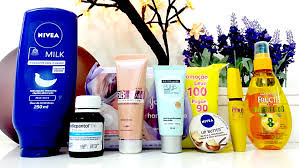The image captures a POV shot from eye level of an array of health and beauty products arranged on a tabletop. Behind the products, two pot plants add a touch of natural decor. The plant on the right, housed in a white pot, features a dark purple to blue flower that resembles the fluffy, petal-like structure of wheat. To the left, a branch adorned with yellow flowers extends out of the frame, adding a splash of color and contrast.

From left to right, the products are organized as follows: A dark blue bottle labeled "Nivea," a small medicine-like cylinder with a white cap, a beige squeeze bottle, another white squeeze bottle, a pack of yellow wipes positioned behind, a tiny spray bottle likely containing perfume, a yellow cylinder, and a clear plastic spray bottle filled with yellow liquid.

The composition is both aesthetically pleasing and functional, showcasing a variety of personal care items against a backdrop of vibrant, blooming plants.